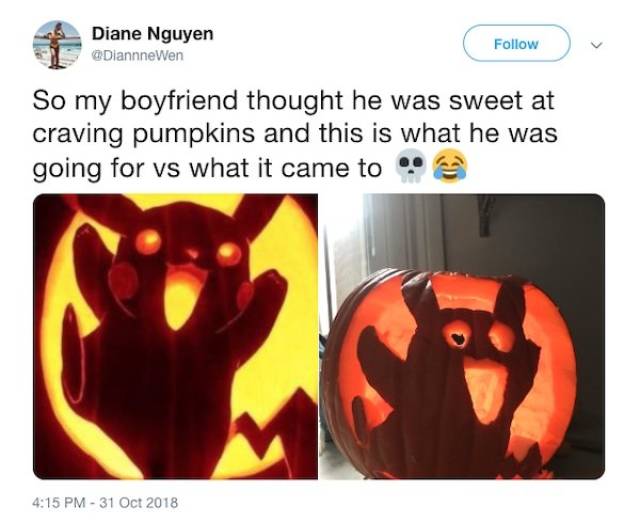In this social media screenshot, the profile belongs to Diane Nguyen, displayed at the top with her handle @DianeNguyen. To the left, there's a circular profile picture that shows Diane standing on a beach in a bikini. On the right, there's a clickable button to follow her, accompanied by a down-pointing caret for more options.

The post humorously shares her boyfriend's attempt at pumpkin carving. Diane captions it with, "So my boyfriend thought he was sweet at carving pumpkins and this is what he was going for versus what it came to," followed by a skull and a laughing emoji. The post then showcases two images side by side. 

On the left, there's a professionally carved pumpkin depicting a character from an animation, brilliantly illuminated with a bright yellow light. The craftsmanship is exceptional, with intricate details that bring the character to life.

On the right is her boyfriend's rendition of the same character. While it's clear he put in effort, the carving doesn’t match the finesse of the original. It’s lit with a softer orange glow and though you can discern the mouth, eyes, and overall shape, it lacks the precision and detail of the reference pumpkin.